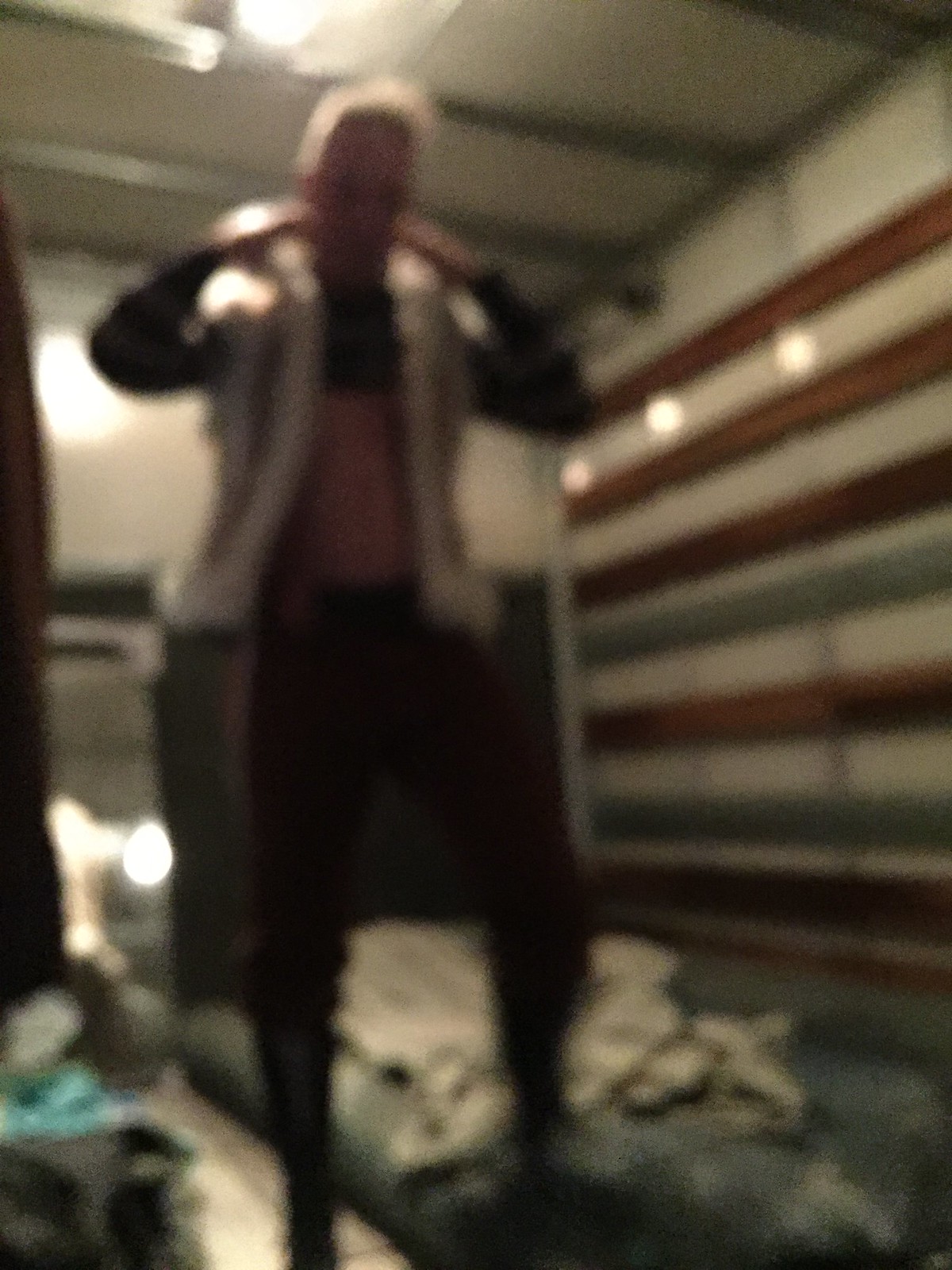The photograph is a blurry, grainy indoor image taken in poor lighting, depicting a person standing just to the left of center, occupying most of the frame from top to bottom. The person appears to be wearing dark pants and a light-colored vest over a long-sleeved crop top or shirt. Due to the blurriness, their facial features are indistinguishable, making it difficult to determine their gender, but they might have short, light-colored hair, possibly blonde, which seems translucent and sticks up slightly.

Their pose is somewhat peculiar; their arms are extended outwards with elbows bent and hands near their cheeks, almost as if they are covering their ears. One leg, likely the left, is propped up on a blue or gray sleeping mat, which also has a bunched-up white blanket on it, while the other leg rests on the floor.

The background features a white ceiling with gray or silver beams and multiple bright lights. The wall behind their right side (left on the image) includes a section with horizontally-aligned boards or possibly metal beams with alternating lines of white, red, and grayish blue. Another part of the wall has vertical wooden panels, suggesting it might be part of a garage door or wall decoration. Additionally, to the left of the person, there's a blue object, perhaps a tarp or cloth, amidst some general clutter. The overall scene is slightly messy and cluttered, enhancing the chaotic feel of the image.